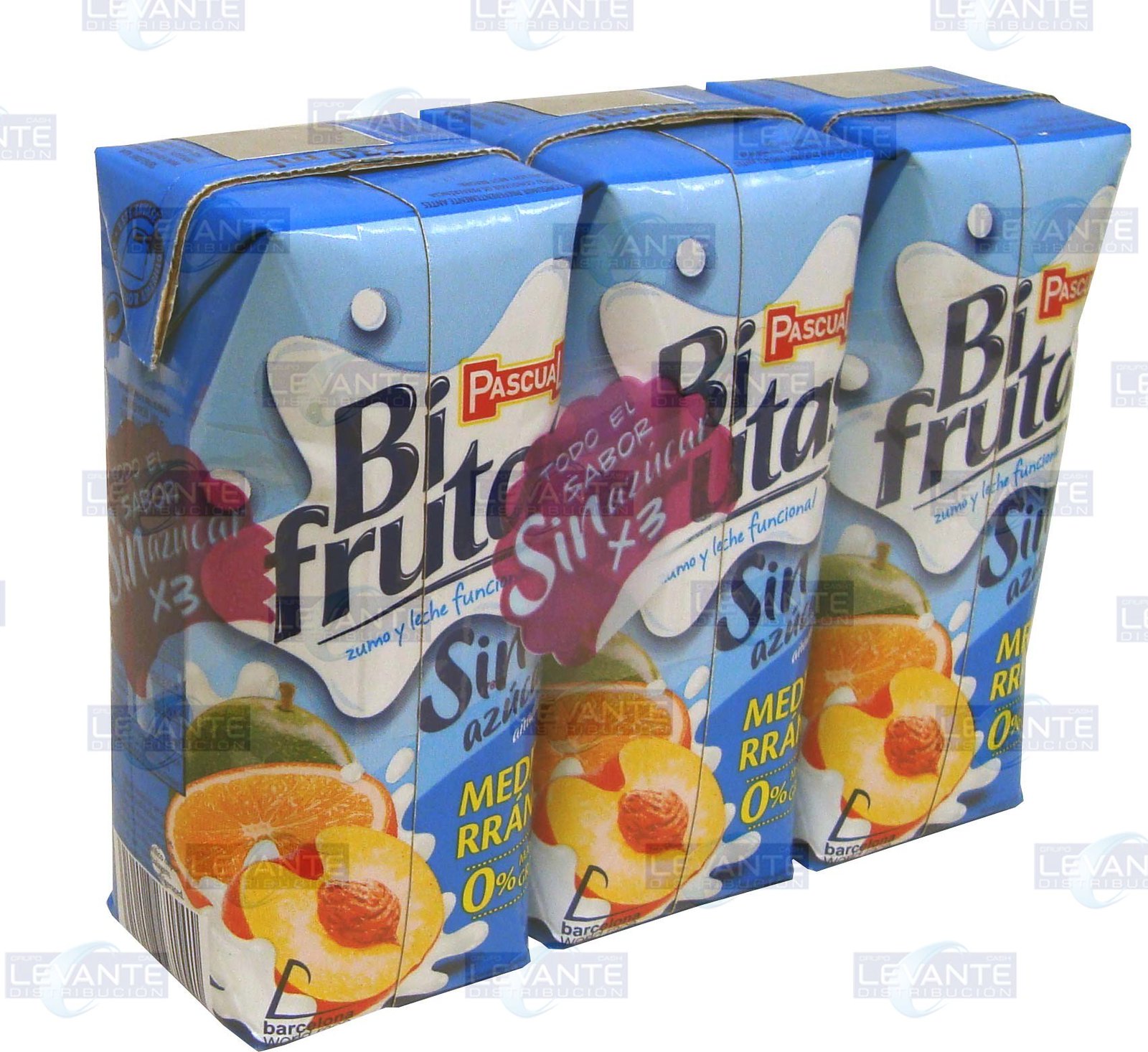This image is a detailed color photograph of three identical juice boxes, arranged next to each other in a straight line and viewed diagonally from the front, facing the bottom right corner. The boxes have dark blue tops and feature a light turquoise color on the front. Each juice box is adorned with images of a halved peach with the pit visible, a sliced orange, and a green apple positioned at the bottom left corner of the box. The label text, in Spanish, prominently reads "BIFRUTA" on the first line, with additional details like "FRUTA," "ZUMO Y LECHE FUNCTIONAL," and "SIN AZUCAR" accompanying it. There is also a "0%" notation, although its specific meaning is unclear. The juice boxes appear to be shrink-wrapped together for display, possibly intended for promotional or illustrative use on platforms like a website. The entire image is set against a white void, lacking any visible background or surface. Overlaid repeatedly across the photograph is a transparent watermark in the form of a blue rectangle, which reads "LEVANTE," with additional, smaller, and illegible text below it.